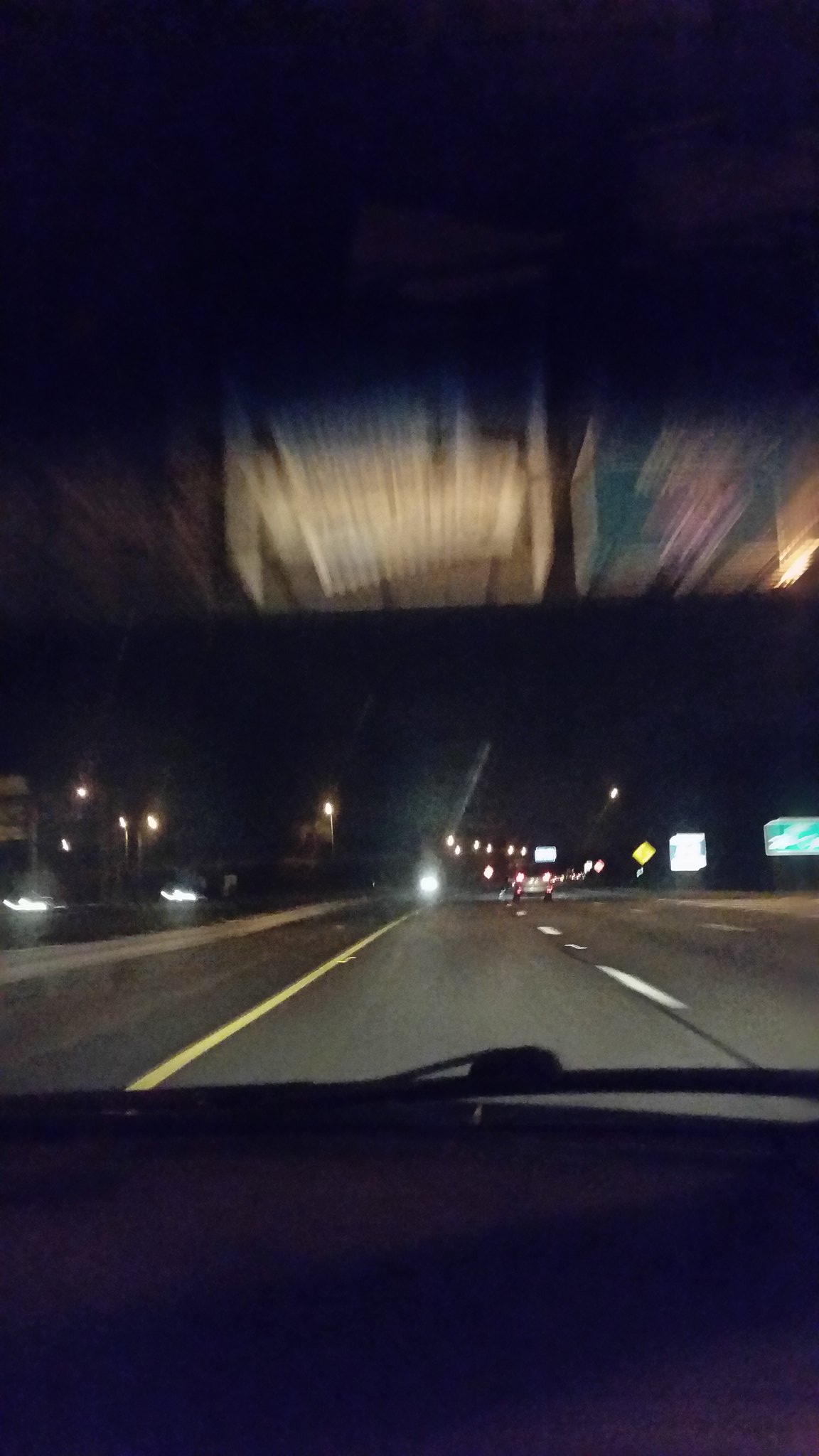A blurry night-time photograph taken from inside a moving vehicle captures a scene on a multi-lane expressway. The image is in portrait orientation, likely shot with a mobile phone. The bottom third of the photo shows the car's dashboard and a windshield wiper resting outside on the windshield. Through the windshield, blurry lights from oncoming vehicles are visible, indicating the car is traveling in the leftmost lane. Road signs are present to the right, including green, white, and yellow ones, though the text is unreadable due to the motion blur. Overhead, directional or informational signs are seen; the left sign appears mostly white, while the right sign is predominantly green with a splash of red or pink in the center.